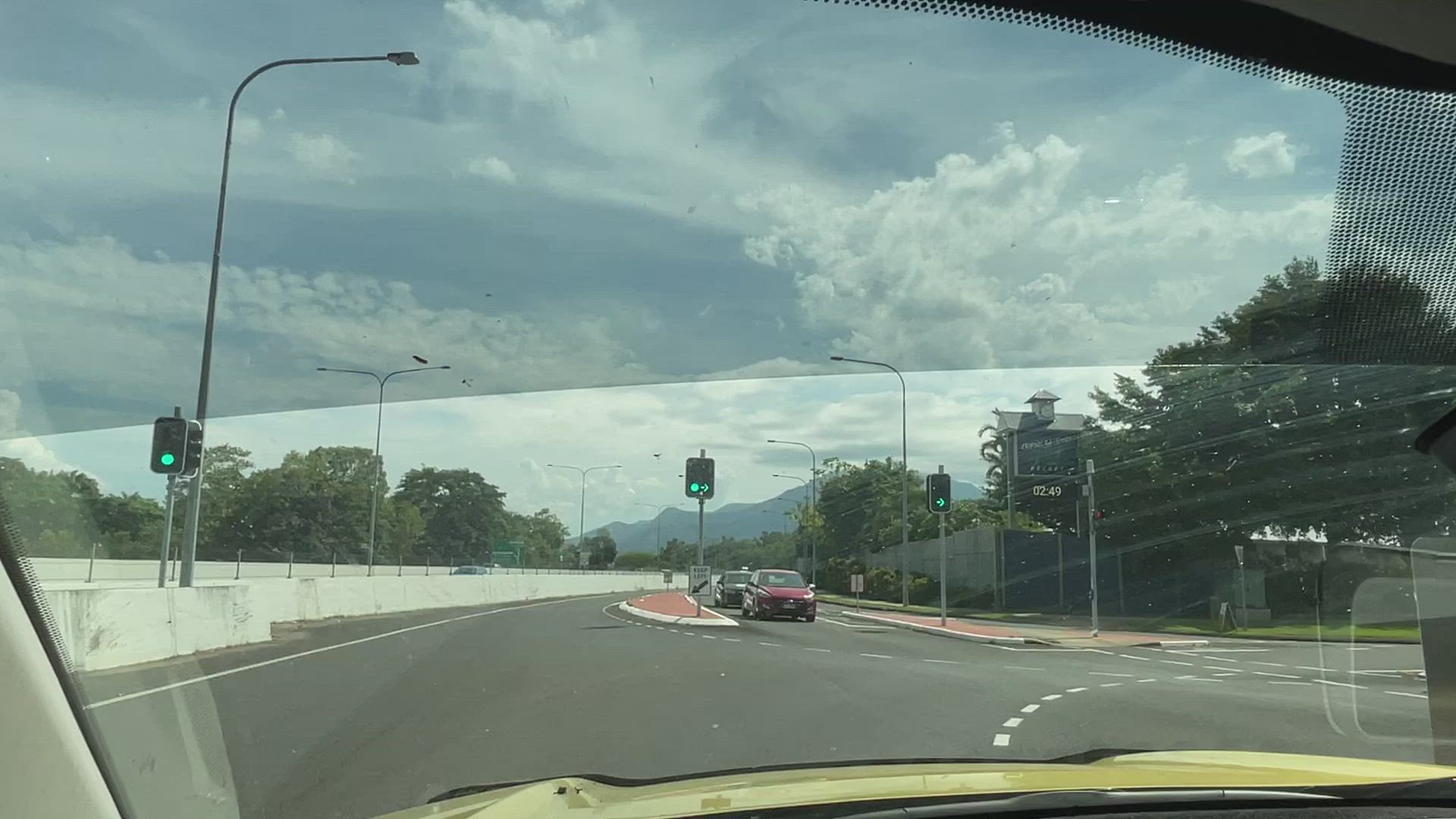The image depicts the view from inside a left-hand drive car, looking through the windshield from the driver’s perspective. The top of the windshield has a greenish-colored sun band, and a strip of clear windshield is visible below it. The lower portion of the windshield shows the road ahead clearly, which includes an off-white dashboard along the bottom. The hood of the car is medium yellow, lighter than a school bus. 

In the center of the view, the roadway curves to the right, marked by a white dotted line. There's a fenced-in area with substantially sized, leafy trees on the right-hand side, as well as a sidewalk along the fence line. Directly across the center of the image, two or three cars are stopped at a traffic light in a brick median section dividing the road. There are three traffic lights visible, all displaying green: one in the brick median, one on the far left corner, and another on the far right. 

The highway is divided, with cement Jersey barriers on the left side extending up to the middle of the photo. In the background are several leafy, rounded trees and a tall residential building near the upper right corner of the image. Mountains are faintly visible, mostly obscured by trees, beneath a blue sky with scattered clouds. The image, characterized by its detailed view of the roadway, traffic signals, and surrounding landscape, suggests a setting indicative of either an American or European highway.